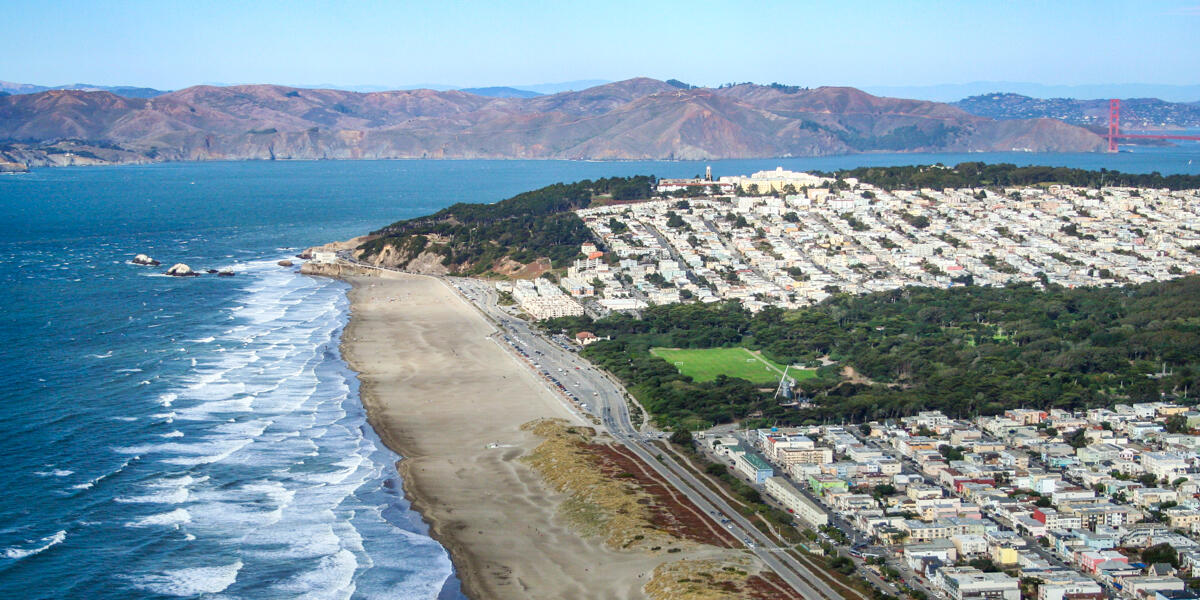This aerial photograph captures a stunning coastal view of San Francisco, prominently featuring the iconic red Golden Gate Bridge in the upper right-hand corner, set against a backdrop of rolling hills and mountains. The scene is divided by an expansive, very green park area, bordered by colorful buildings in shades of pink, aqua, and yellow. These structures line neatly organized streets on both sides. A long, sandy beach stretches across the center towards the left, with vibrant blue water lapping at the shore, creating lots of white foamy waves as they crash. A highway runs parallel to this beach, where a few cars are visible. The water appears to wrap around the town, emphasizing the picturesque quality of the coastal inlet. The sky is a clear, bright blue, suggesting the photo was taken during the daytime. The overall atmosphere of the image conveys a peaceful yet vibrant coastal city with a distinctive harmony between urban development and natural beauty.